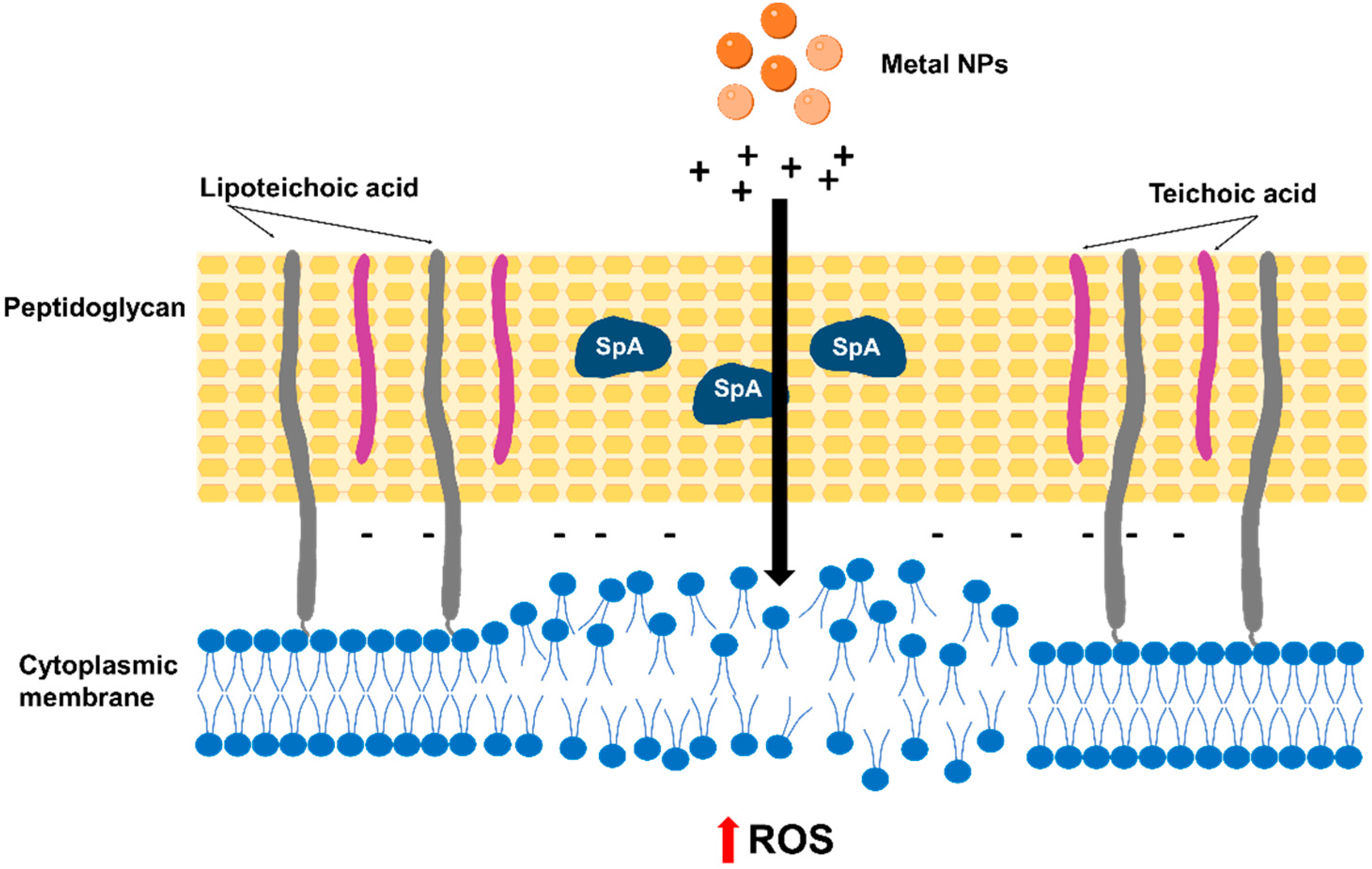The diagram illustrates a biological or chemical process, starting at the top with orange spheres labeled "Metal NPs." Below these spheres are black plus signs, followed by a downward-pointing black arrow. This arrow penetrates a yellow barrier labeled "Peptidoglycan," which also contains gray lines labeled "Lipoteichoic Acid" and additional lines labeled "Teichoic Acid." Furthermore, within the yellow barrier, there are blue blobs marked "SPA." Beneath this yellow layer lies a blue barrier composed of two rows of blue spheres with small protruding lines, labeled "Cytoplasmic Membrane." At the diagram's base, the letters "ROS" are labeled in black atop a red upward-pointing arrow, directing attention back towards the blue circles above them.